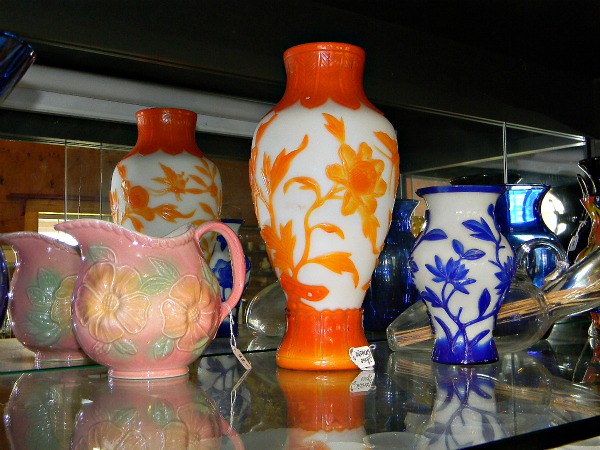This photo captures an indoor setting bathed in sunlight shining through a window in the background, revealing a wooden wall. The ceiling features a fluorescent light fixture that spans from the upper left corner to the right, with two unlit bulbs. Below, there is a highly reflective glass or mirrored shelf that vividly mirrors the collection of ornate ceramic vases arranged on it.

To the left of the image is a large, pink ceramic jug adorned with yellow and green 3D embossed flowers and an elegant handle for pouring. Next to it stands a tall, slender vase, distinguished by its bright orange and white design. This vase is narrow at both the base and the top, with a broader middle section, featuring orange flowers and leaves painted along its white surface. To the right, there’s a smaller, similarly shaped vase, showcasing blue flowers and leaves on a white body, with blue glazed sections at the top and bottom. Behind these main vases lies a clear vessel partially visible, possibly containing straw or grass stems, adding to the intricate arrangement. The vibrant ceramic items, some with tags, reflect beautifully off the mirrored and glass surfaces, creating an almost kaleidoscopic effect.